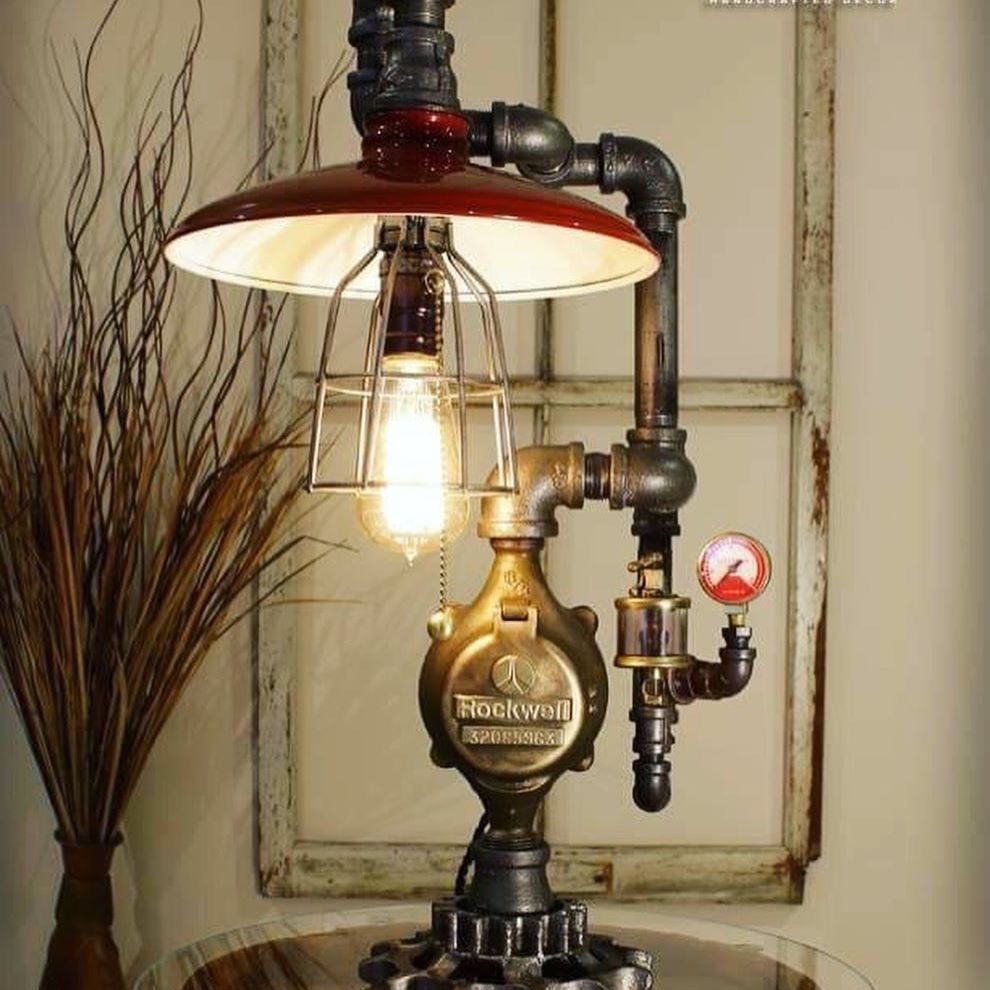The image depicts a striking steampunk-inspired lamp art piece, constructed from an intricate arrangement of metal pipes and gears. Situated at the base is a vintage round glass table, evoking an industrial aesthetic. Central to the artwork is a substantial metal gear, topped with a round pipe piece inscribed with "Rockwell" and a series of numbers. From this base, a curved pipe extends to the right, connecting with another vertical pipe. This section features a red and white gauge protruding to the right. Ascending further, the pipe system includes several curved segments, one of which terminates in a large black metal component. Hanging from this component is a burgundy red lampshade with a white interior, beneath which is the light fixture. The bulb is encased in a protective copper-colored metal cage, with a gold pull string dangling below for operation. Completing the scene, a rustic window frame with no glass leans against the wall in the background, and a vase with decorative hay adds a touch of homely charm to the left of the image. The entire piece exudes a vintage, industrial flair, reminiscent of the 1930s or 1940s.